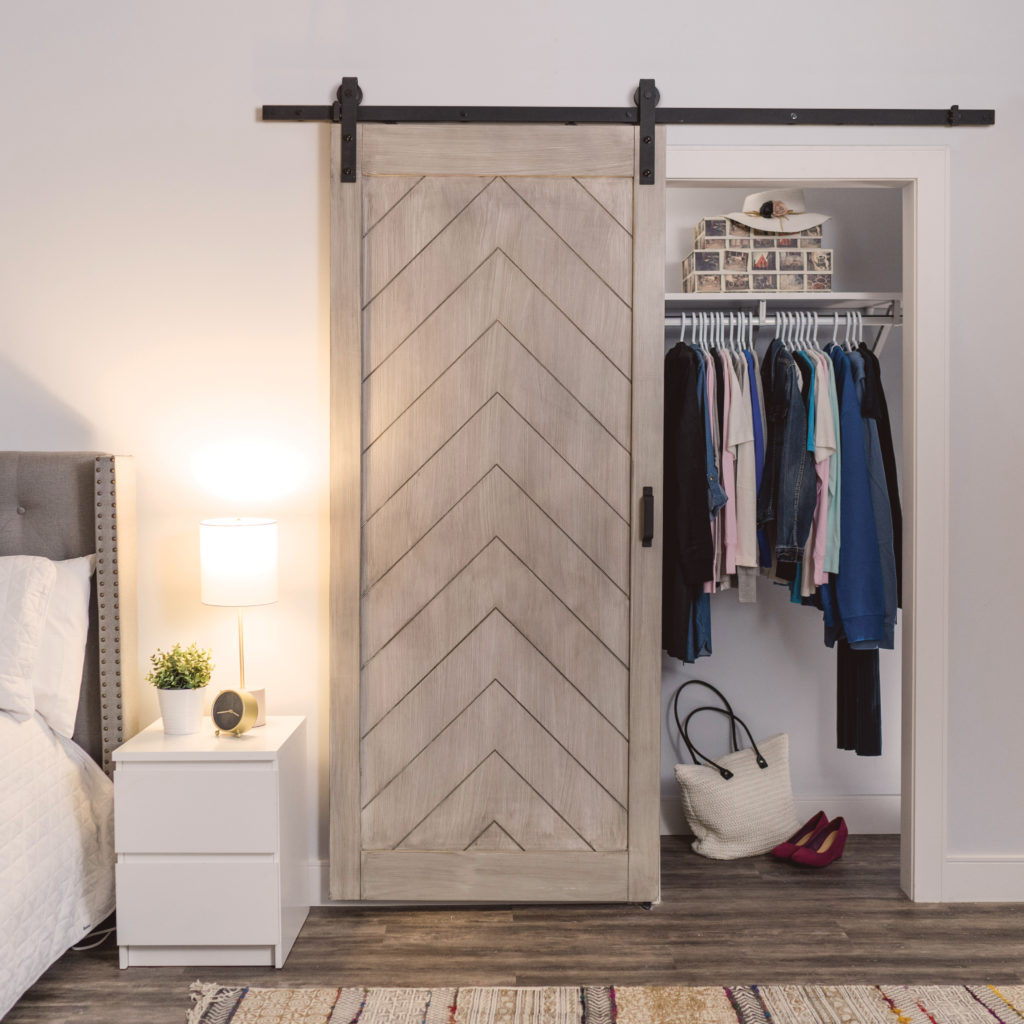The image is a detailed indoor photograph featuring a distinctive, open sliding barn-style closet door subtly crafted from light beige wood with a vertical chevron pattern. The door hangs on a black metal rail spanning the doorway, equipped with rollers that allow it to slide open and closed. In front of the closet, we see a light gray wall complemented by white baseboards and trims. Inside the closet, clothes hang neatly from a rack, with a pair of burgundy high heels and a white tote bag with black handles on the floor. Above the hanging clothes, there’s a shelf holding keepsake boxes and a hat. 

To the left side of the image, partially in frame, is a cozy bed adorned with a white bedspread, white pillow, and a gray headboard. Beside the bed, there's a small white nightstand with two drawers, topped with a potted green plant, a turned-on lamp, and a gold clock. The flooring is a rich dark brown wood that extends seamlessly into the closet area, adding a warm, cohesive touch to the room. Additionally, a long rectangular rug with vertical stripes in shades of white, blue, and red rests atop the elegant wooden floor, adding a layer of style and vibrancy to the setting.